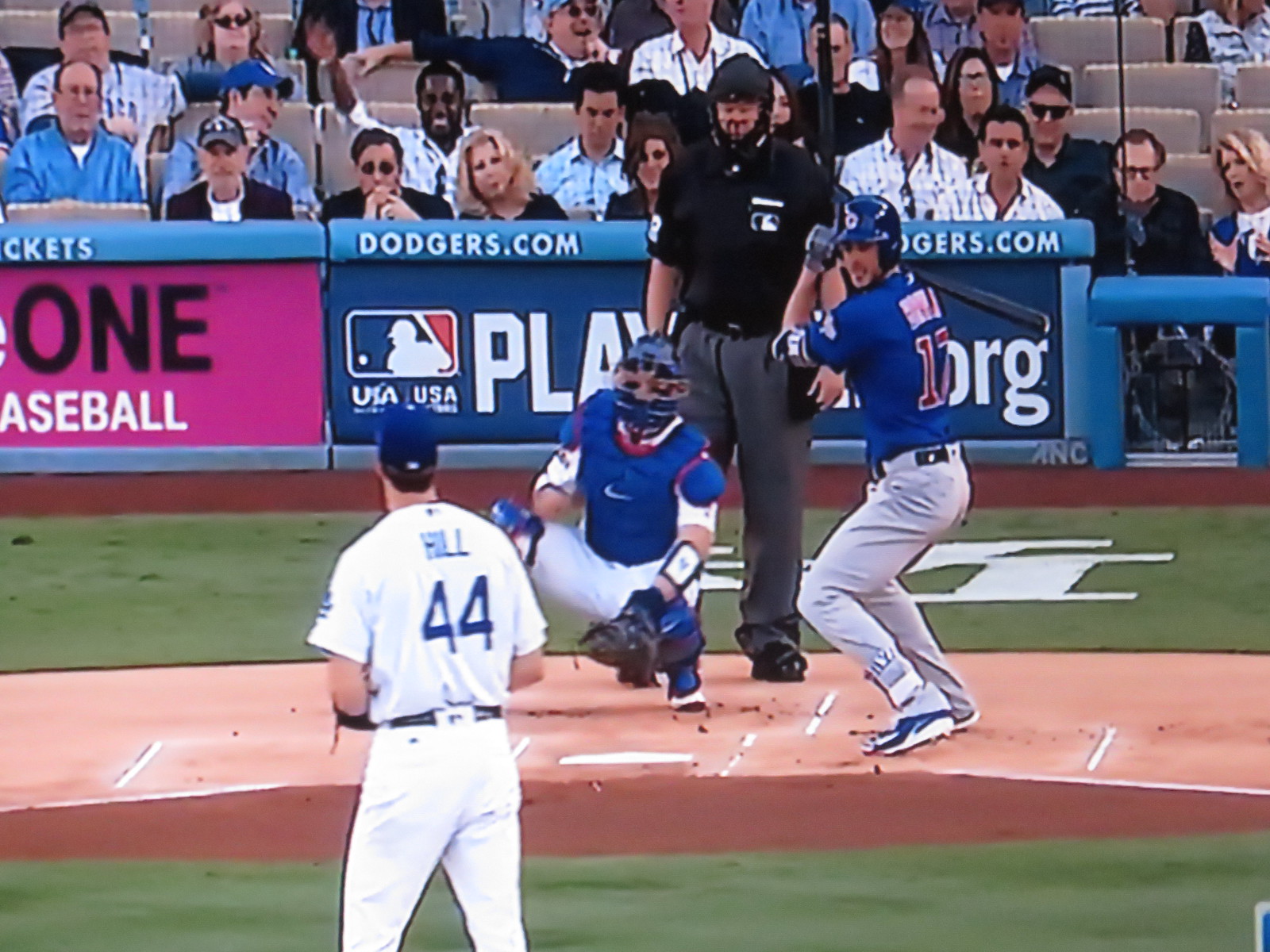This image captures a daytime Major League Baseball game from a vantage point just behind the pitcher on the mound, focused on the action at home plate. At the bottom left of the screen, the pitcher, number 44 Hill, stands outfitted in a white uniform with blue lettering and a blue cap. He appears to be concentrating on the batter, catcher, and umpire situated directly in front of him in the center of the image. The catcher, kneeling behind home plate, is dressed in white with a blue protective vest, while the umpire, positioned behind him, wears a black face mask, short-sleeved shirt, and dark gray long pants. The batter is identified by his blue jersey with red lettering and gray pants, donning a helmet featuring a circular logo with a wing, indicative of the Cleveland Indians. The field is surrounded by fans seated behind a safety net, and the wall behind them displays the text "Dodgers.com." The scene, set in a baseball park under the clear daylight, vividly showcases the game's intensity and anticipation.